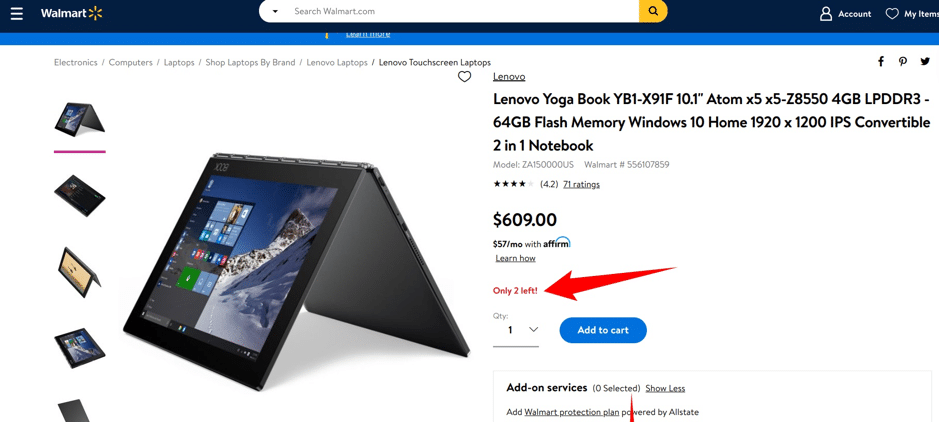This image displays a Walmart webpage with a distinct black border at the top and a light blue strip at the bottom. On the top left corner, there are three horizontal lines stacked atop one another, commonly known as the menu icon. Adjacent to this icon is the Walmart logo. Centrally placed on the top navigation bar is a white search bar highlighted by a yellow magnifying glass icon. To the right of the search bar, there are options labeled "Account" and "My Items."

Directly underneath these options, on the left side, is a section dedicated to electronics, featuring categories such as "Electronics," "Computers," "Laptops," "Shop Laptop by Brand," "Lenovo Laptop," and "Lenovo Touchscreen Laptops." On the far right of this section, social media icons for Facebook, Pinterest, and Twitter are displayed.

Beneath this navigation area, there is detailed information about a specific product: the Lenovo Yoga Book YB1-X91F. Key specifications of this product are highlighted, including a 10.1-inch display, an Atom X5-78550 processor, 4GB of LPDDR3 RAM, 64GB of flash memory, and Windows 10 Home operating system. The screen resolution is noted as 1920 x 1200 pixels, and the device is described as a convertible 2-in-1 notebook with an IPS display.